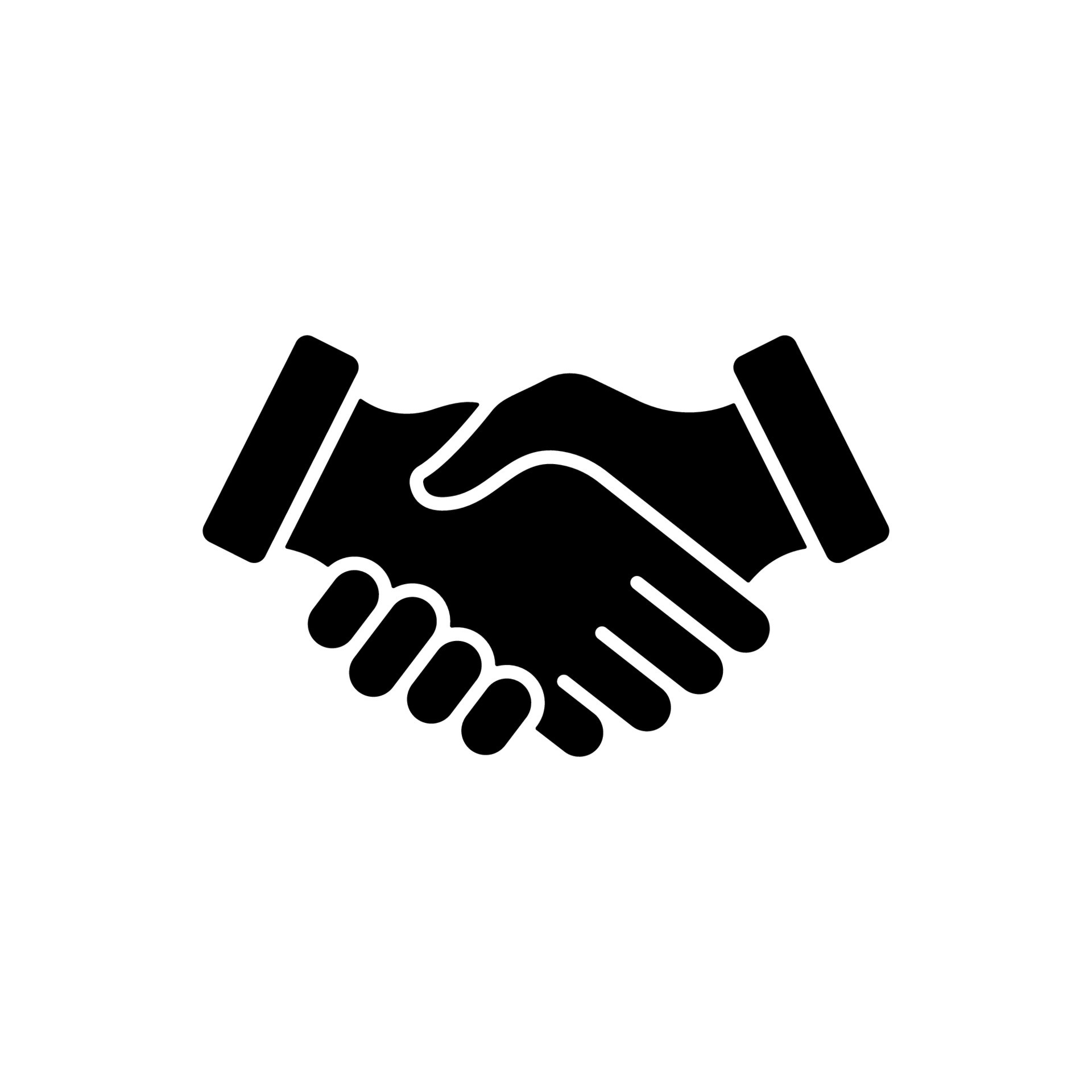The image features a minimalist black and white depiction of two hands shaking, drawn with digital precision. The background is entirely white, enhancing the simplicity and focus on the hand gesture. Both hands are rendered in black, extending from the wrists where they are marked by black bands resembling shirt cuffs. One hand displays all four of its fingers up to the knuckles, while the other hand is partially hidden behind, showing the thumb and fingertips wrapping around. The composition is symmetrical, with both cuffs oriented diagonally, adding a balanced and professional appearance to the handshake. No other elements are present in the image, emphasizing the pure, straightforward nature of this illustrative handshake.